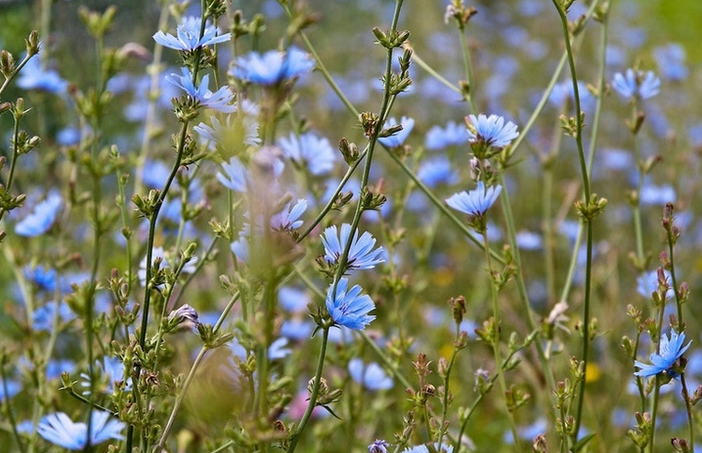This close-up snapshot captures a dense and prolific cluster of wild blue chicory in vibrant detail. The slender green stems of these wildflowers are adorned with several tiny buds and blossom profusely, showcasing blue petals that range in color from pale blue to sky blue, with square-tipped ends, giving each flower a uniform appearance. The blossoms are open wide around a pale yellow center, creating a striking contrast. The stems feature tiny joints from which new buds sprout, with some flowers fully bloomed and others in varying stages of opening. The image conveys a lush field of these chicory flowers, with additional blooms extending into the blurry background. In the upper right-hand corner, the scene is framed by the limbs and leaves of a tree, adding a touch of surrounding greenery to the predominantly blue and green palette of the photograph.